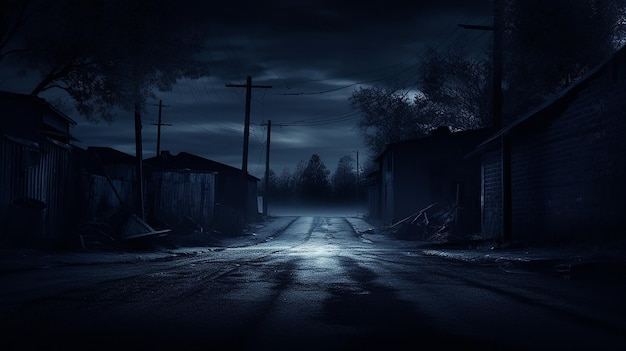The image, possibly a painting or a digital print, depicts a nighttime scene dominated by dark and light shades of blues and blacks. The rectangular artwork, roughly five inches wide by three inches high, showcases a somewhat eerie alleyway or old road. The ground appears paved and slightly wet, reflecting the subtle illumination around the area. On the left side, dilapidated houses and rickety fences line the road, accompanied by telephone or electrical poles that create a cross-like silhouette, possibly hinting at an ominous or cursed atmosphere.

The right side of the image features shrubs and trees interspersed between more old buildings. The road begins wider at the bottom and narrows as it leads into the distance, flanked by shadowy, dense trees that might suggest a dark forest. The center of the composition is highlighted by a burst of moonlight, casting a whitish glow on the road, creating a striking contrast against the overall dark palette.